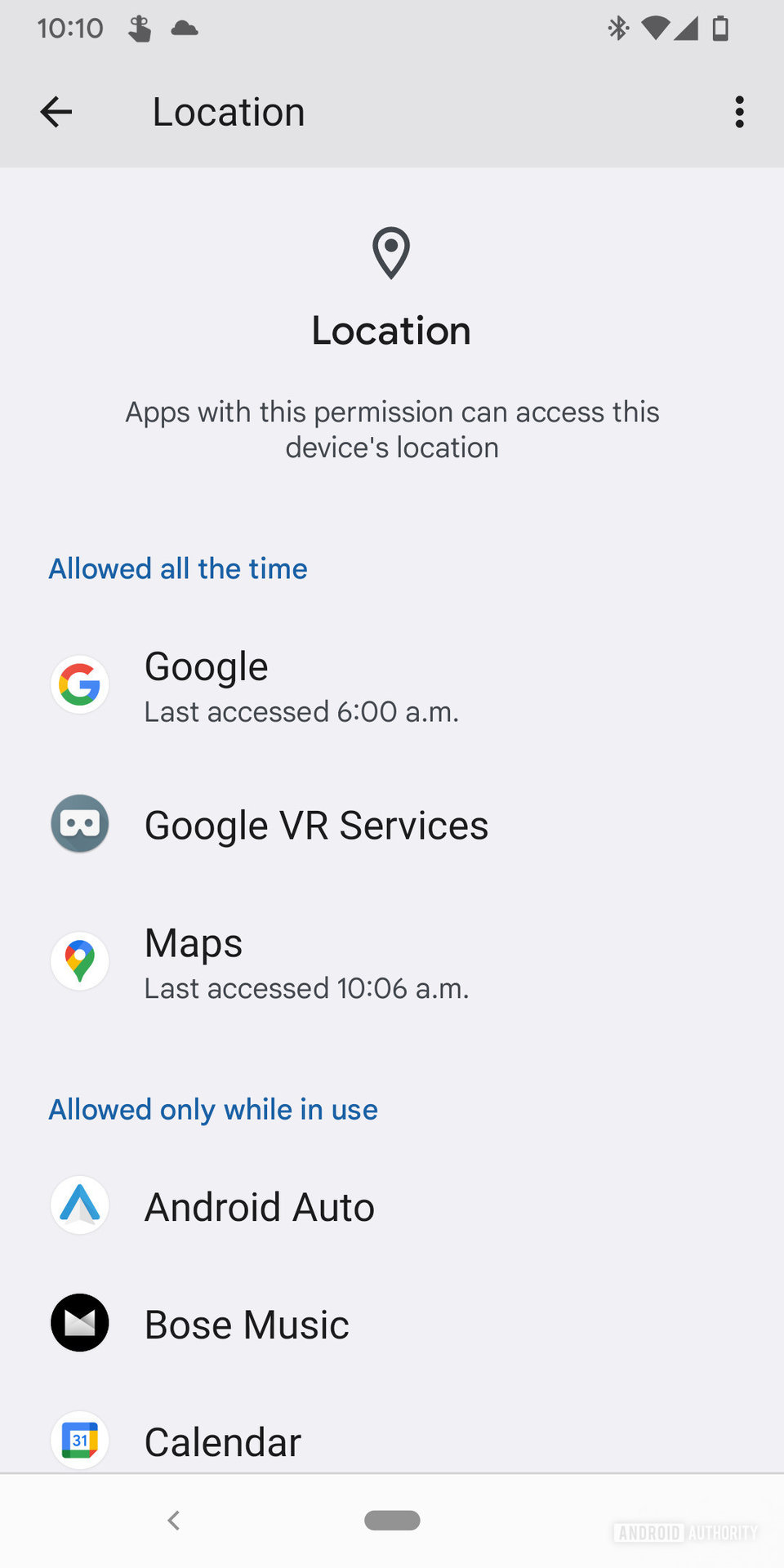This image is a screenshot captured from a cell phone, showcasing the device's 'Location' settings panel. Positioned at the top left corner, the panel is labeled 'Location' with a pincushion icon immediately above it. Directly below, the text states, "Apps with this permission can access this device's location."

The interface is divided into two sections. The first section, titled "Allowed all the time" in small blue letters on the left, lists three apps: Google, Google VR Services, and Maps. Each app is accompanied by information about the last time it accessed the device's location: "Google - last accessed at 6:00 AM," "Maps - last accessed at 10:06 AM."

The second section, labeled "Allowed only while in use," includes apps such as Android Auto, Bose Music, and Calendar. The screenshot cuts off the list, suggesting more entries could be seen by scrolling further.

In addition to the location settings, the screenshot captures essential phone status icons at the top left, displaying the current time along with Wi-Fi, Bluetooth, phone signal strength, and battery percentage indicators.